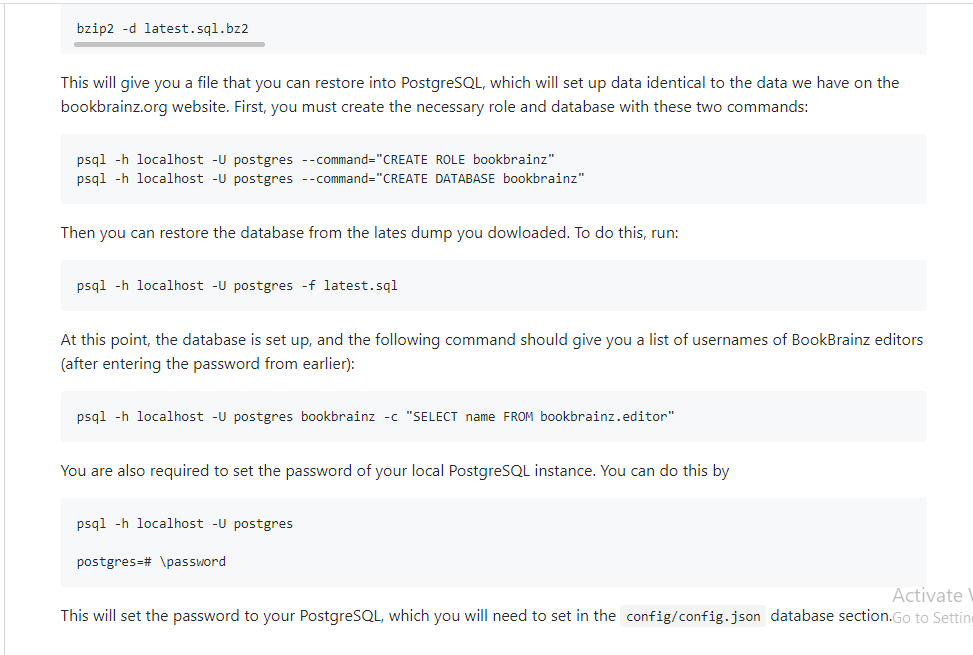In the image, the focal point revolves around coding, specifically database management using PostgreSQL. At the top left corner, there's a statement that reads "bzip2-d latest.sql.bz2", followed by a gray horizontal line and a concise description. The description outlines the process of obtaining a file that can be restored into PostgreSQL to replicate the data present on the bookbrains.org website. It instructs users to create the necessary role and database with two specified commands. Below this, there's a separate area listing these commands. Following this, another section advises users to restore the database from a recently downloaded dump by running the command "psql -h localhost -U postgres -f latest.sql".

The middle-left portion of the image states that once the database is set up, executing a particular command will yield a list of usernames of bookbrain editors, assuming you've input the password created earlier. Beneath this, there’s a command prompt illustration for initiating the search. The final note in the image emphasizes the need to set the password for the local PostgreSQL instance. The visual presentation and instructional text work harmoniously, guiding users step-by-step through the database restoration and setup process.